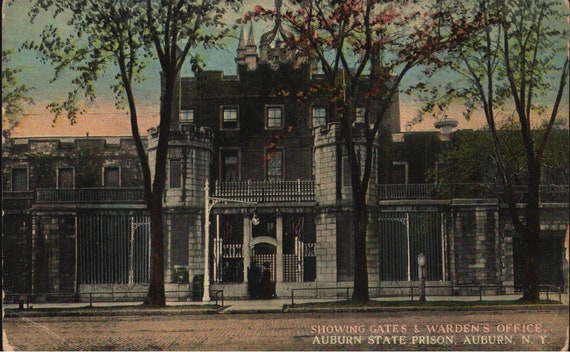This is a vintage photograph of Auburn State Prison in Auburn, New York, depicting an imposing and ornate structure that resembles a black castle. The front gate, which also has a castle-like appearance with two security towers flanking the entrance, is composed of dark gray metal with accents of gray and white. Standing in front of this gate are four tall trees, two with green leaves and one with red leaves, located along a tree-lined road. The streets in front appear to be made of bricks or cobblestones, with short metal railings encircling the grassy areas where the trees are planted. A streetlight is positioned before the gate, directing illumination toward the entrance. The building itself, a four-story structure made from white or possibly brownstone bricks, features a central taller section with lower walls on either side. The photograph, taken in late afternoon, captures bright blue skies adorned with white clouds and an orange streak indicating a setting sun. In the bottom right corner, white text reads "Showing Gates and Warden's Office, Auburn State Prison, Auburn, New York," adding context to the historical scene.